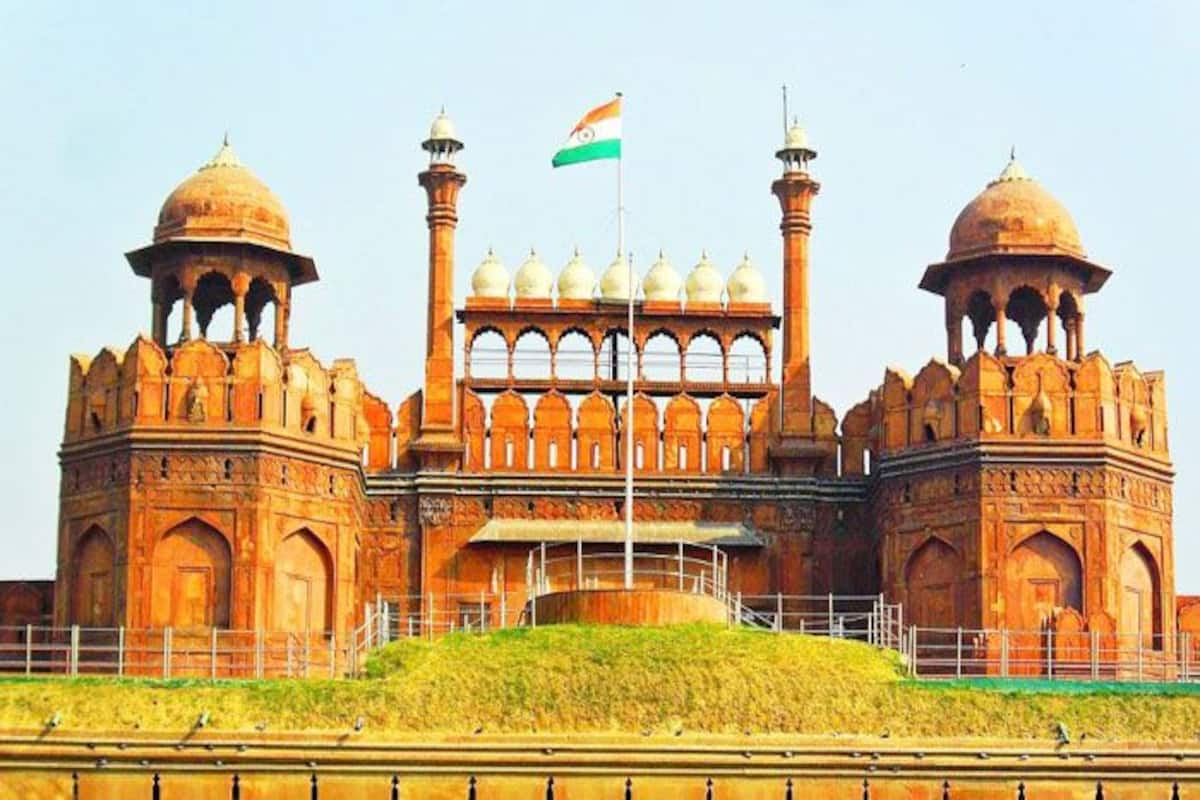The image is a photograph taken outdoors during the daytime, depicting a large, reddish-brown stone fort with a light blue sky in the background. The central structure features a flat wall, which is an orangish color resembling brick or stone and has seven white domes on top. Dominating both the left and right sides of the fort are two identical, wide, circular towers that have domed tops and bear some resemblance to military fortifications. Inside these larger towers are thinner towers capped with white domes. The middle section of the fort includes a large flagpole from which the Indian flag, colored green, white, and orange, is flying prominently. A round stair railing descends from this central area to both the right and left. Surrounding the fort is a grassy area, possibly a fortified encampment with defensive capabilities, enclosed by a silver fence. The overall scene suggests a blend of architectural symmetry and historical significance, set against the serene backdrop of a clear sky.